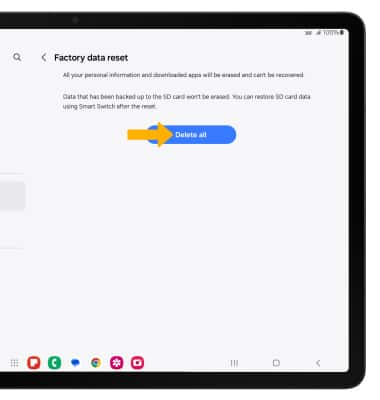This image, captured from a device screen, displays a factory data reset prompt. The top of the screen showcases a magnifying glass icon against a white background. In bold black text, the message "Factory Data Reset" is prominently featured. Below, a detailed sentence warns, "All your personal information and apps will be erased and can't be recovered." Additionally, it notes, "Data that has been backed up to the SD card won't be erased. You can retrieve SD card data using Smart Switch after the reset."

A blue button labeled "Delete All," with the text in white, is highlighted by a digital yellow arrow pointing directly at it. The image appears to be slightly cropped, revealing a black border running from the top around the right side and partially over to the left. At the bottom of the screen, one can also spot various icons, though their details are not fully visible.